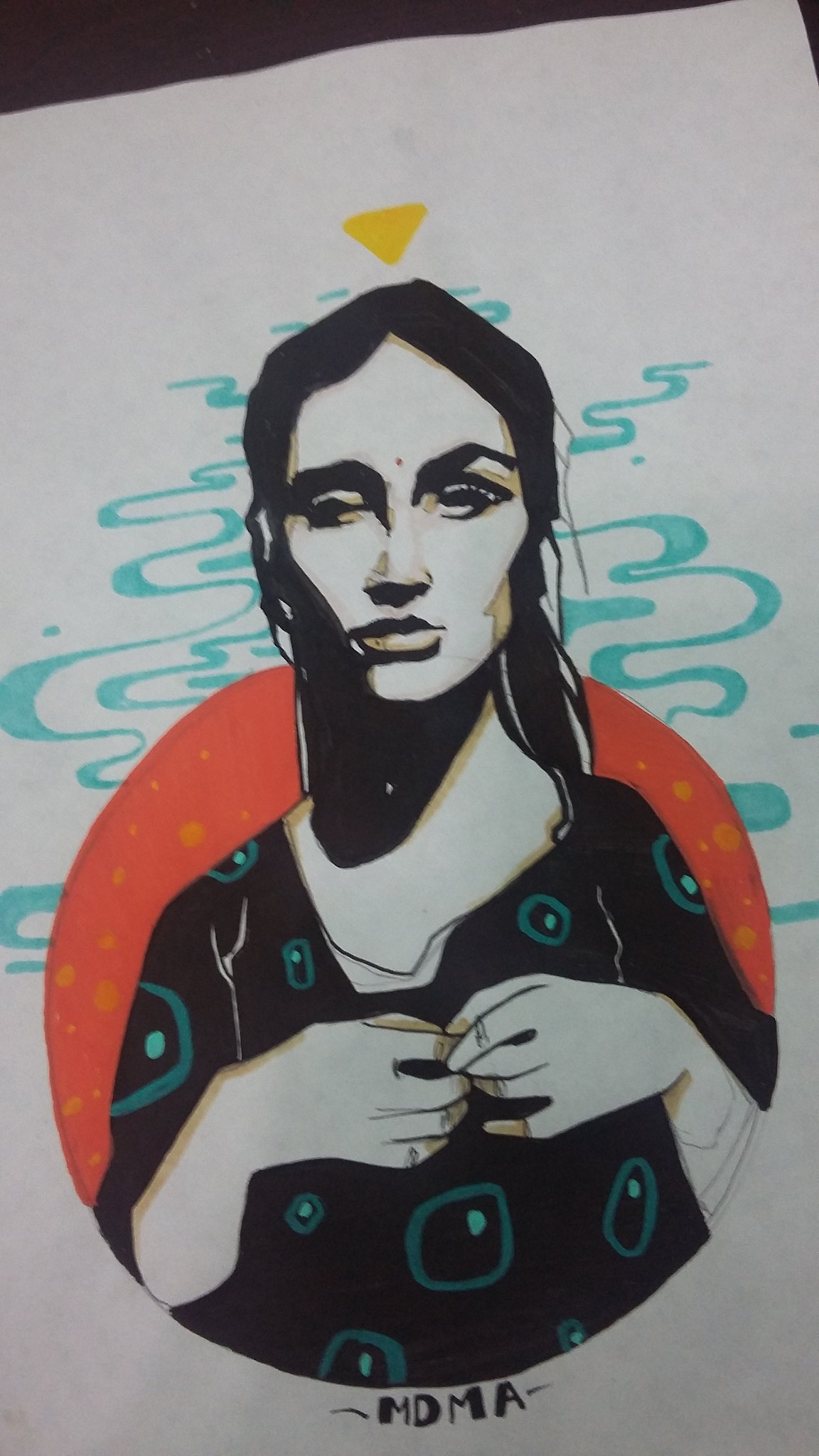This detailed color photograph captures a vibrant piece of art likely displayed indoors on a flat surface, possibly concrete. The artwork appears to be a mural or a highly stylized painting of a woman, depicted in a cartoonish style. She has long, dark, and somewhat messy hair pulled back, with thick eyebrows and a slightly off-centered eye, suggesting a lazy eye. A prominent red dot is located between her eyes.

The woman is wearing a black dress covered with blue squares that have rounded corners and light blue dots in their upper right corners. Her hands are delicately held together at the fingertips, positioned in front of her chest. Surrounding her head and shoulders is a bold red circle with yellow dots, resembling a sun.

The background is adorned with aqua or green squiggly lines, evoking the motion of water or smoke. At the top of the image, there is a black triangle with a piece of white paper placed on it. An inverted yellow triangle hovers just above her head, adding another layer of geometric complexity to the piece.

At the bottom of the image, in elegant black script, the word "MDMA" is written, though one source mentioned it as "Mona," suggesting variations or potential confusion in the transcription of the name. Overall, this visually intricate image combines vivid colors, detailed patterns, and whimsical design elements to create a striking, memorable work of art.